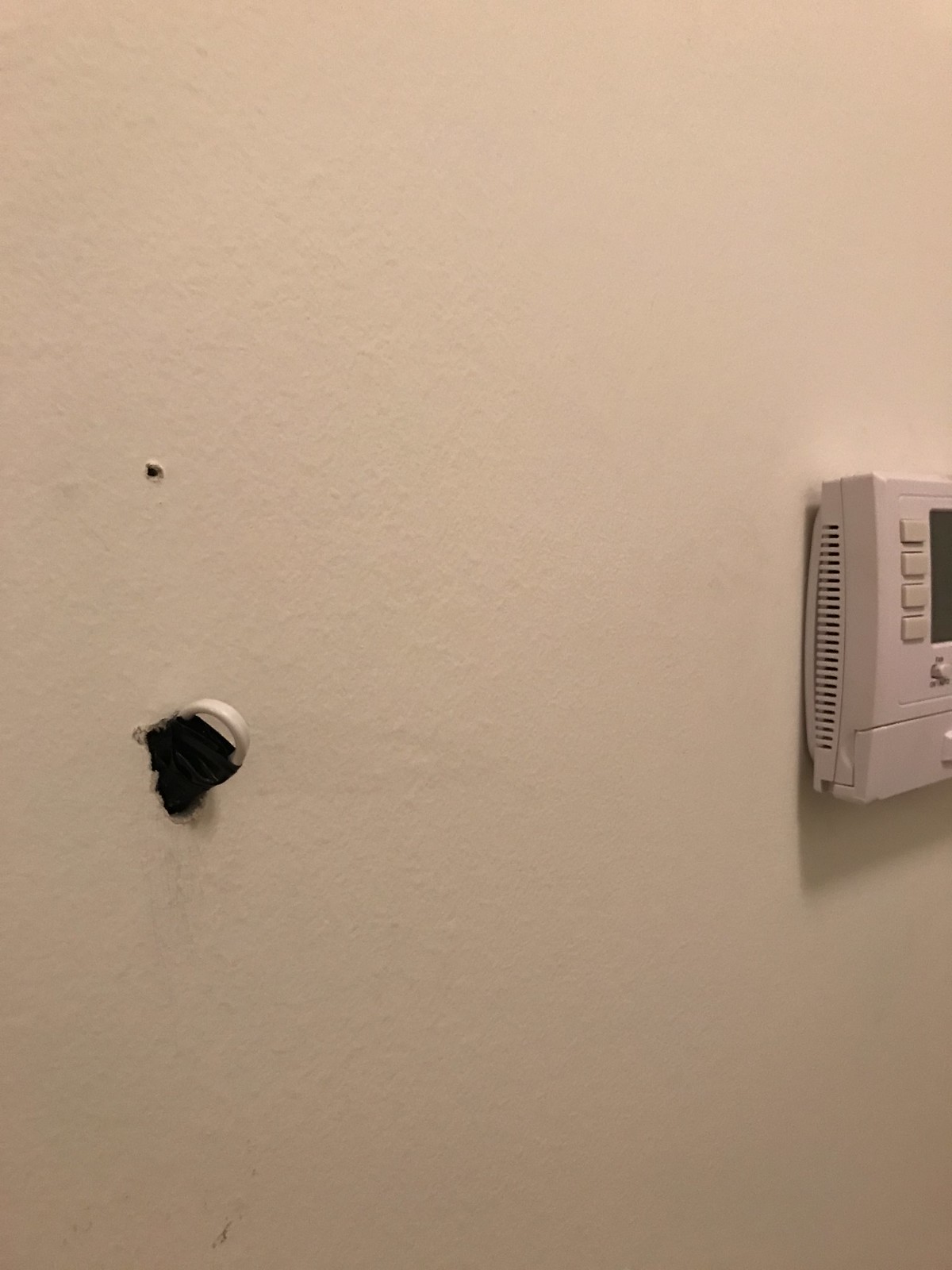The image showcases a textured tan wall, which features an intercom system mounted prominently. The intercom, colored gray, is situated towards the right of the image and appears lighter in texture compared to the rest of the wall. The intercom includes a screen and four buttons, and emits a small amount of light upwards.

Adjacent to the intercom is an object that appears black and slightly resembles a hairnet, held in place by a half-moon-shaped plastic ring. This object initially seemed to be a hole, but closer inspection reveals it is attached to the wall. Above this object, another small mark or indentation can be seen, contributing to the wall’s textured and uneven surface.

The wall itself varies in texture, showcasing ripples and unevenness, with patches of darker tan hues scattered across. The lower left-hand section of the wall appears dirtier than the rest. 

Overall, the visual interest is centered on the interplay between the smooth and rough textures of the wall and the technological presence of the intercom system.